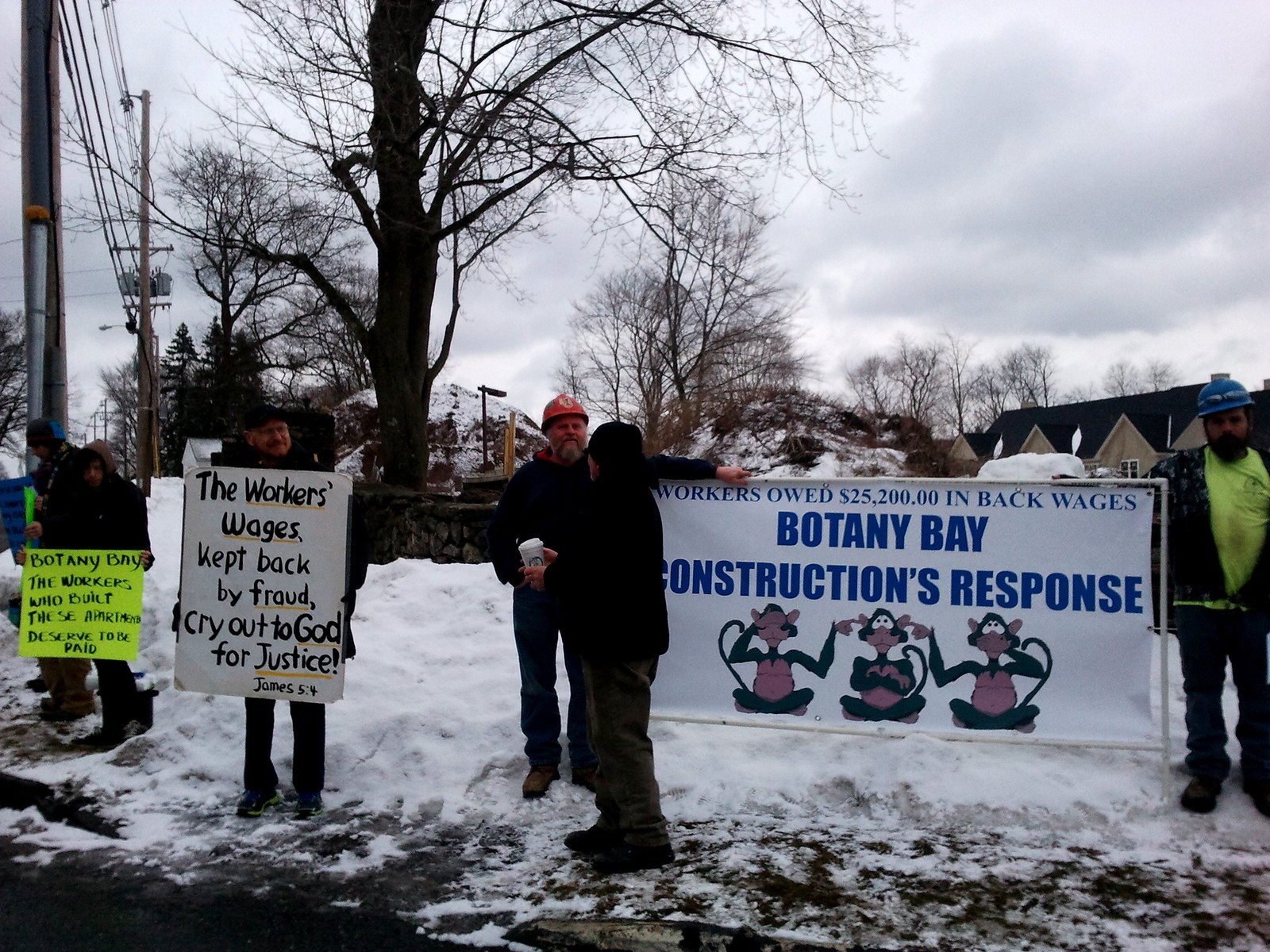In a snowy, leafless landscape, a group of construction workers stages a picket line against Botany Bay Construction for owed back wages. At the forefront, two workers, one in a red hard hat and another in a blue hard hat, hold a prominent white sign adorned with three monkeys representing "See No Evil, Hear No Evil, Speak No Evil." The sign reads: "Workers owed $25,200 in back wages, Botany Bay Construction's response." Slightly to the left stands a man with a black hat holding a white sign that proclaims, "The workers' wages kept back by fraud cry out to God for justice." Adjacent to him, at the left edge, another protester in a fluorescent yellow-green shirt holds a similarly passionate sign stating, "Botany Bay: the workers who built these apartments deserve to be paid." The group, appearing determined despite the cold, stands near a leafless tree under a gray, overcast sky.